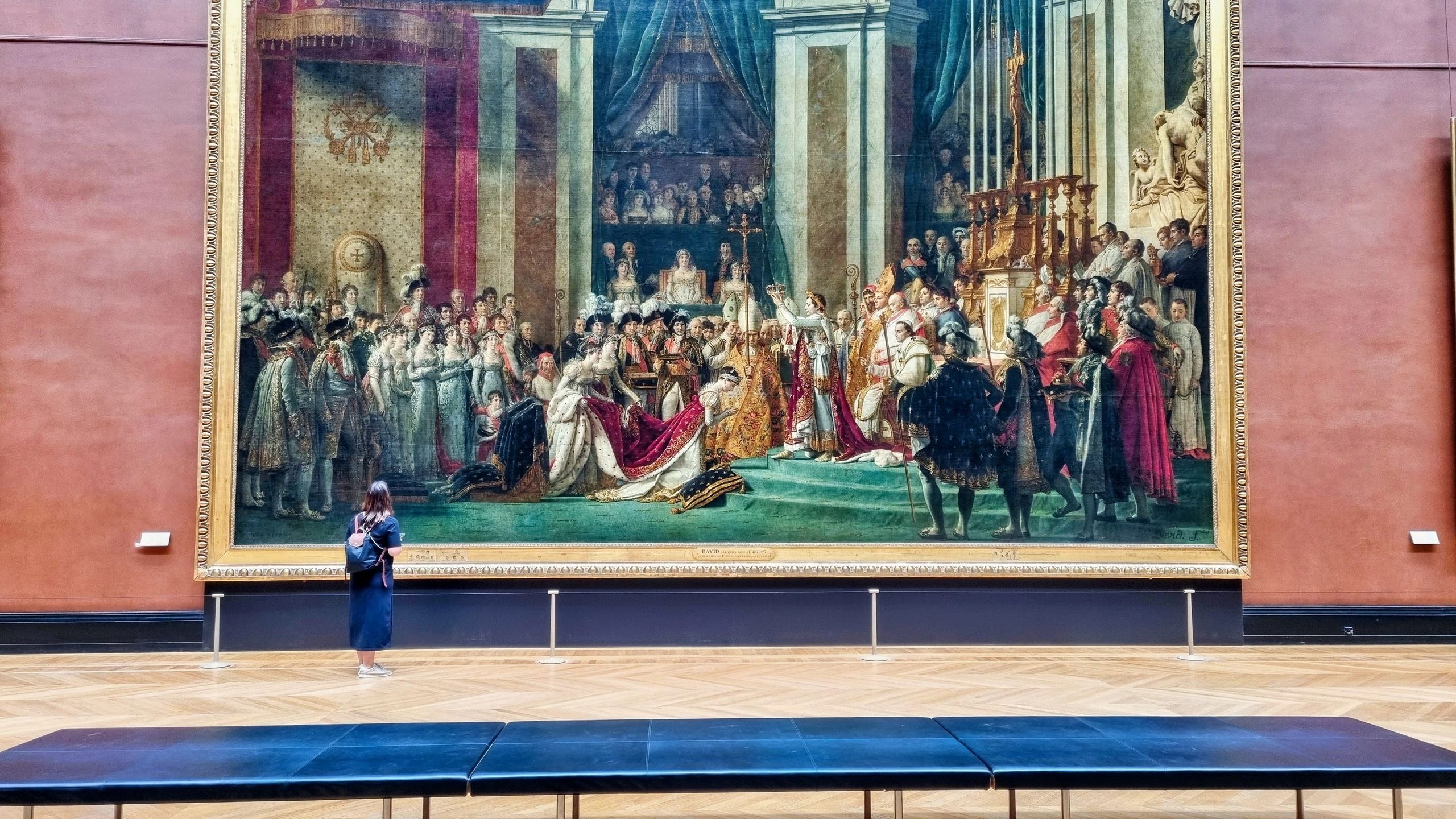In this image, a girl wearing a long blue gown and white canvas shoes is standing in front of a large painting, entirely engrossed. She carries a black and brown backpack and is positioned in a spacious room with a terracotta-colored wall. The wall features a massive painting in a gilded, ornately carved gold frame. The painting depicts the coronation of Napoleon, with intricate details such as a green-carpeted stage, dignitaries in elaborate robes, including the Catholic Church officials, and a grand altar with a cross. Josephine is seen kneeling on a few steps as Napoleon prepares to crown her, surrounded by an audience of royals and nobles in elaborate attire. The room also contains a table and black benches for visitors. The impressive scale of the painting makes the girl appear very small in comparison.